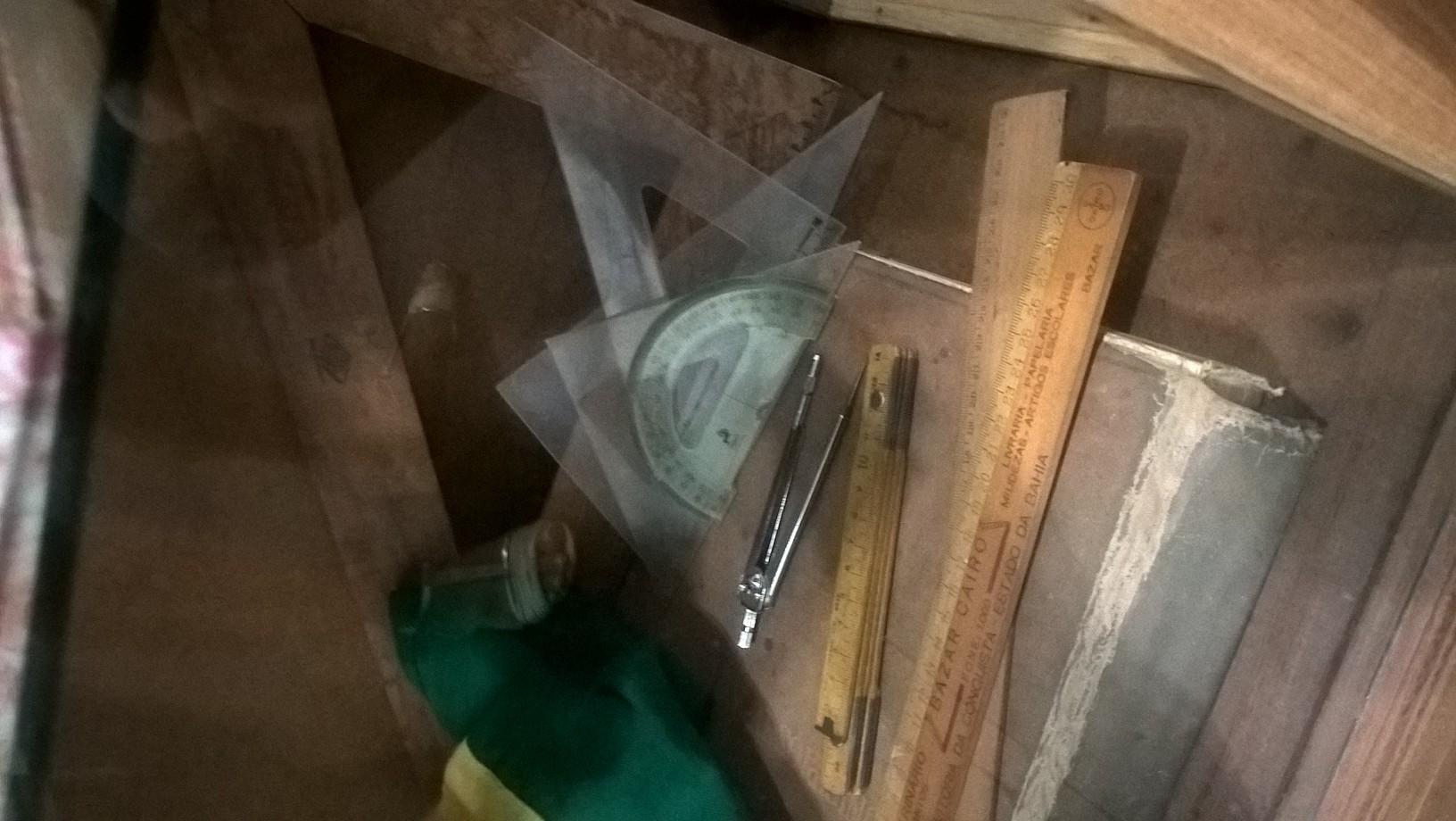The image depicts an array of mathematical and geometrical tools scattered underneath what appears to be a desk or enclosed within a wooden case, possibly in a workshop setting. The assortment includes three aged and slightly dirty rulers, a half-circle protractor for measuring angles, and a metal compass resembling a wishbone, designed for drawing perfect circles. Additional measuring devices, such as squares and other protractors, are also visible. To the left, there is a green and yellow bag or garment. These items are encased in glass, as evidenced by reflections visible in the image—one showing the photographer, who has dark hair and light skin, in the upper right-hand corner, and another of feet on the glass surface. The surrounding wood appears to be processed, adding to the workshop ambiance.